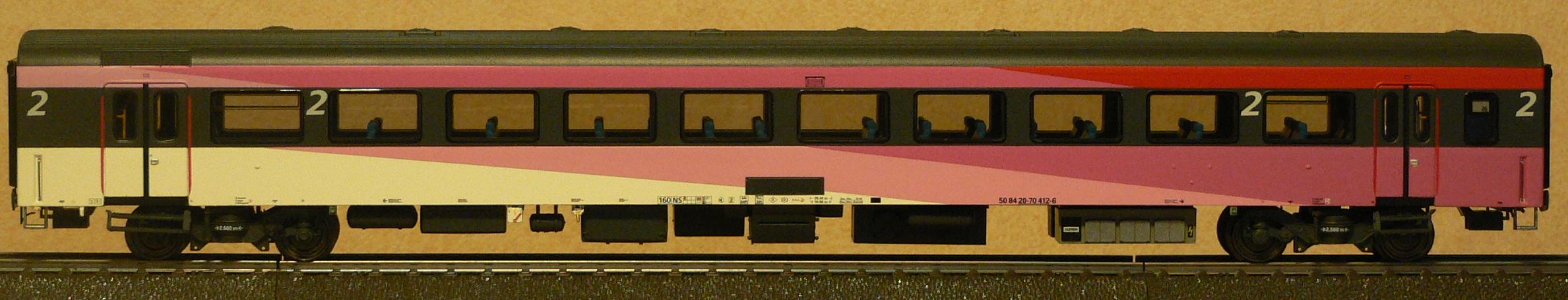This image depicts a long, narrow illustration of a vibrant train car, distinct from an engine compartment or caboose. The colorful vehicle occupies the majority of the rectangular scene, standing on black wheels set against lightly detailed pebbled ground, hinting at a railway bed. Yellowish-brown surrounds frame the background, emphasizing the train car’s dominance in the composition.

The vehicle's upper section features a brown or black rounded roof, beneath which a red stripe runs just above a series of windows. Below these windows, the body is adorned with diagonal patterned stripes transitioning from yellow to light red, and then to darker red hues. Noteworthy is the recurring number "2" displayed in four locations, positioned at both the front and back of the train car. These distinctive elements combine to create a vividly colorful and detailed depiction of a train car on tracks.